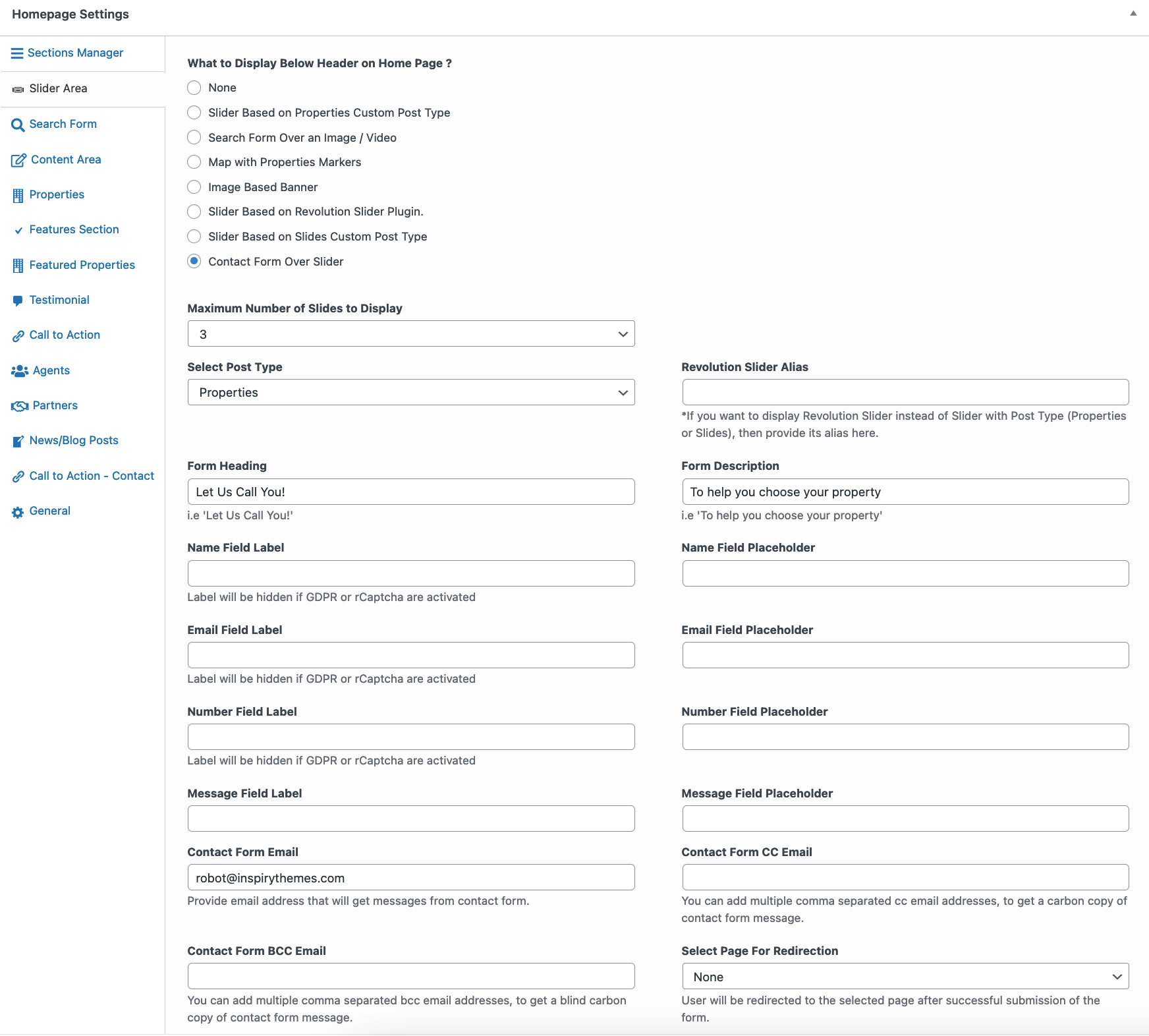The screenshot depicts a website's backend interface for configuring the homepage settings. In the upper left corner, the page title "Home Page Settings" is displayed in black text. Just beneath this heading, a vertical navigation menu extends from the top to the bottom of the screen, featuring various sections in blue text, including "Manager," "Search Form," "Content Area," "Properties," "Features Section," "Featured Properties," "Testimonial," "Call to Action," "Agents," "Partners," "News Blog Posts," "Call to Action," "Contact," and "General." Each navigation item is accompanied by its corresponding icon, enhancing visual guidance.

On the right side of the screen, a form is visible, stipulating settings related to the display below the header on the homepage. The form includes a dropdown menu to select the maximum number of slides to display, another dropdown menu for selecting the post type, and a heading field. Below these settings, a text box reads "Let us call you," suggesting a section intended for collecting potential client contact information or similar user interactions. This form is an essential tool for administrators to manage and customize the homepage layout and functionality efficiently.